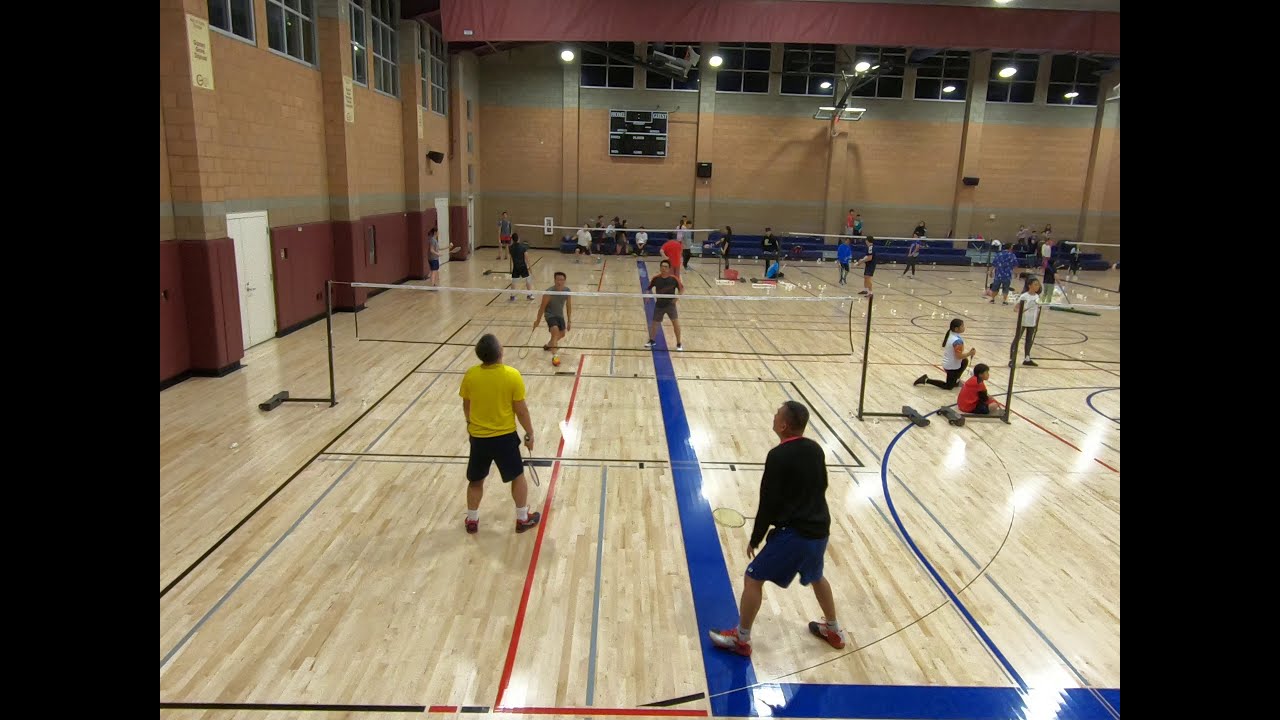The photograph captures the interior of a large, beautifully marked gymnasium flooring, showcasing multiple sports courts delineated by black, gray, red, and thick blue lines. The walls are adorned with a mix of red, dark red, light red, and earthy green stripes, and windows line the top for natural light. The main focus is on an active badminton session where five nets stretch across the hardwood floor, held up by black poles with white trim at the top. There may be a sixth net just out of the frame to the right. Young Asian players, in varied attire—from black sleeve shirts with blue shorts to yellow shirts with black shorts—are engaged in doubles matches, each pair enthusiastically battling it out. A scoreboard hangs on the far wall, and basketball hoops are tilted upwards to make room for the badminton games. Observers, likely younger viewers, sit around the periphery, adding to the lively atmosphere. The gym's multifunctional design and vibrant scene suggest it could be located in China or Japan.